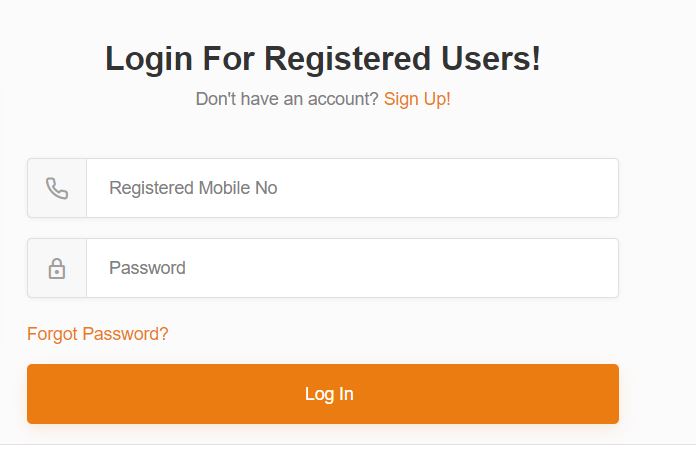The image depicts a minimalist login page with a light gray background and straightforward design, devoid of any photos. At the top-center of the page, the heading "Login for Registered Users" is prominently displayed in large black text. Below this header, there's a prompt in smaller text stating “Don't have an account?” followed by a clickable orange text, “Sign Up”.

Further down, there are two horizontally aligned rectangular text boxes, each not spanning the full width of the page. The first text box contains an icon of a telephone on the far left and the placeholder text “Registered Mobile No.”. Below this, there is another text box featuring a locked padlock icon on the far left, with the placeholder text “Password”.

Beneath these input fields, there is a line of text in orange, reading “Forgot Password”. Concluding the form, at the bottom of the page, is a large orange rectangular button with white, centered text that reads “Login”.